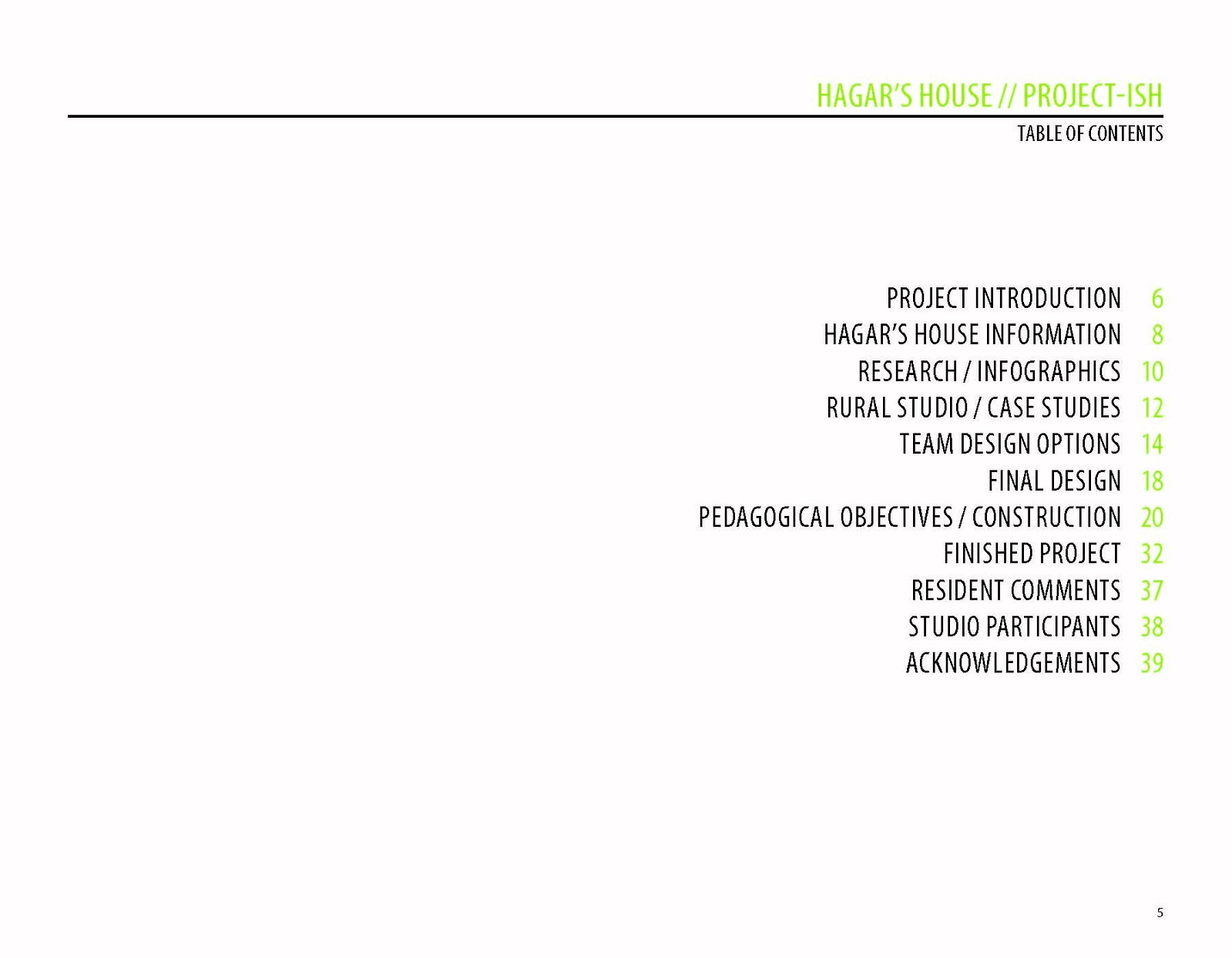The image is a detailed picture of the table of contents from the front of a book or project report titled "Hager's House // Project-ish." The text is predominantly right-aligned with headings and page numbers clearly listed. The top right corner of the page features the project title "Hager's House // Project-ish" in light green on a white background, separated from the rest of the content by a single line. Below the title, in small black letters, it says "Table of Contents." The entries are as follows: "Project Introduction" on page 6, "Hager's House Information" on page 8, "Research/Infographics" on page 10, "Rural Studio/Case Studies" on page 12, "Team Design Options" on page 14, "Final Design" on page 18, "Pedagogical Objectives/Construction" on page 20, "Finished Project" on page 32, "Resident Comments" on page 37, "Studio Participants" on page 38, and "Acknowledgements" on page 39. The entire visual is rendered in black, white, and lime green colors, giving it a crisp and modern look.